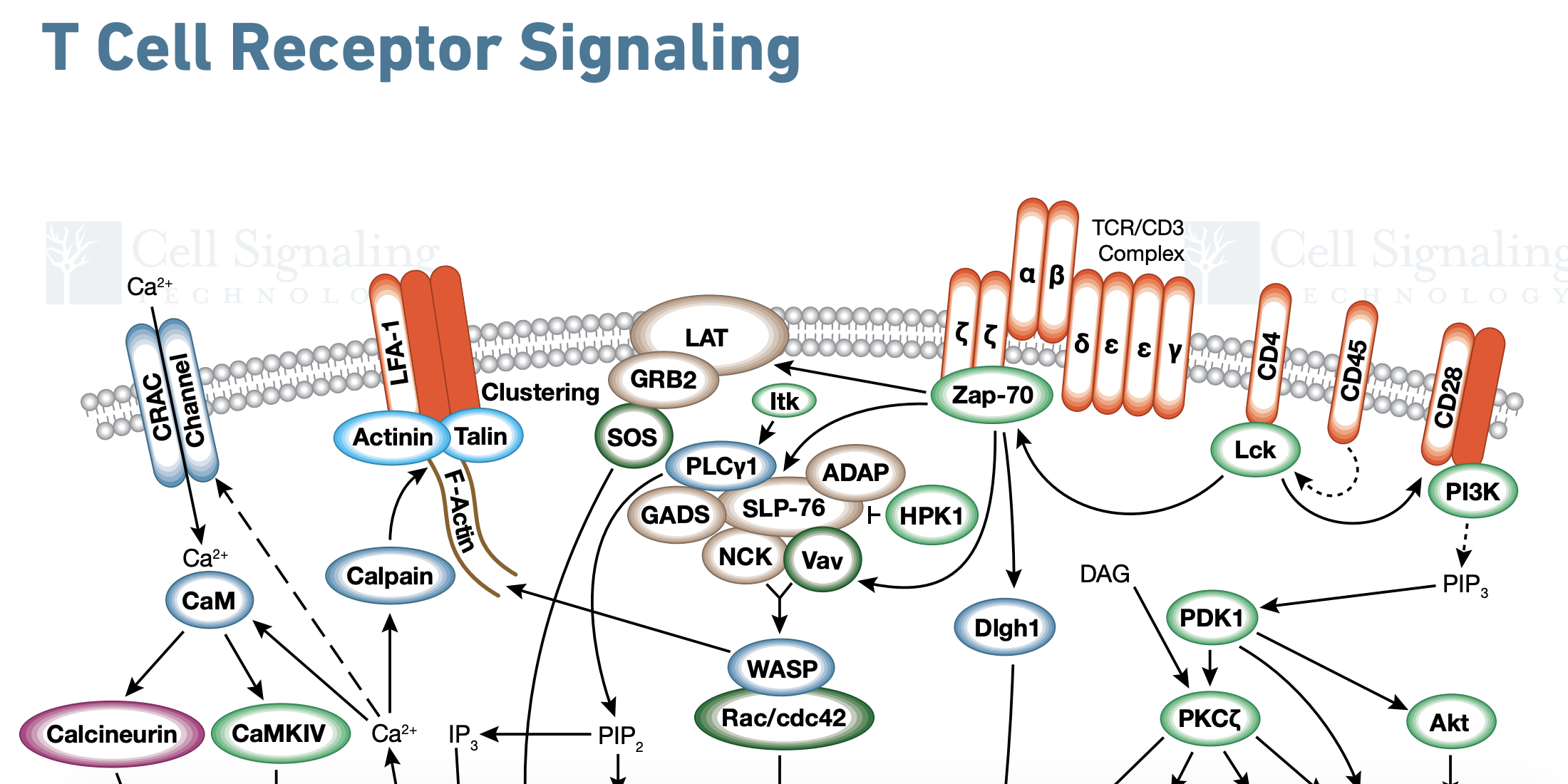This detailed and comprehensive illustration titled "T Cell Receptor Signaling" presents a complex scientific diagram with a transparent background. Displayed prominently in large blue letters at the top is the title "T cell receptor signaling." Both the top right and the left corners feature transparent logos from Cell Signaling Technology. The diagram comprises various colored circles and ovals interconnected with arrows to depict the signaling pathways of T cell receptors.

Specifically, the circles are in shades of green, blue, red, purple, and a lighter purple, each containing scientific abbreviations and labels. For instance, the labels CA, CRAC channel, CAM, calcium neuron, and K, CA, MKIV are highlighted with respective arrows guiding the flow of the signaling process. Additionally, orange circles labeled LFA-1 link to other components with arrows, while a sideway capsule labeled LAT connects through links and arrows to other parts of the diagram. Furthermore, Greek letters denote additional labels, forming intricate connections across eight points, arranged two on the first level, two above them, and four at the topmost layer, emphasizing the layered complexity and interconnectivity of the signaling network depicted.